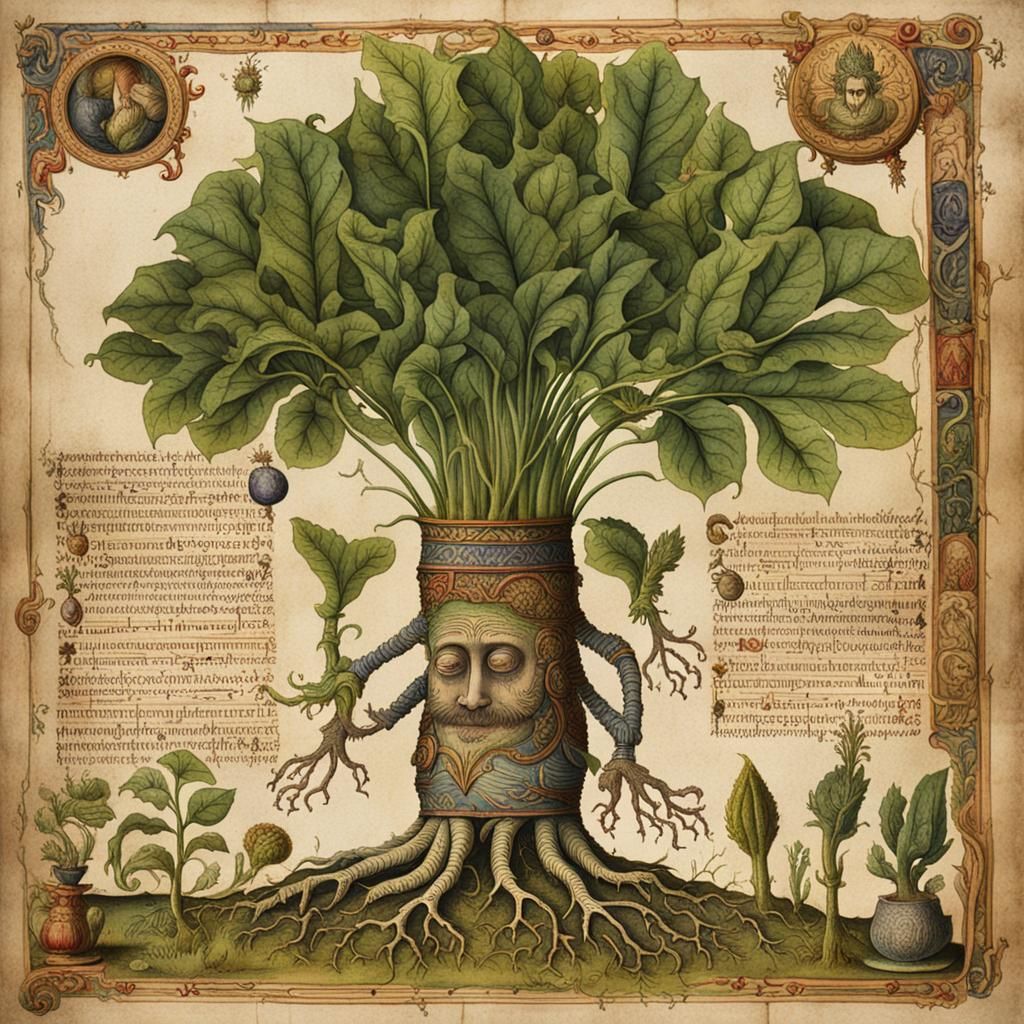This detailed and complex illustration, possibly from a book, features an anthropomorphic tree-like creature set against an earth-toned background. The illustration centers on a tree with roots visibly sinking into a green ground. The tree trunk has a band, resembling a German Stein, and at its center is a human face with large eyes, a narrow nose, and a prominent mustache stretching side-to-side. The face has closed eyes, and a beard extends from the face as well. 

From each side of the trunk extend arms depicted as blue tendrils that transform into brown tree-branch fingers. Above the head, lush green leaves sprout upward, larger than the rest of the creature's body, resembling the expansive foliage of a maple tree.

Surrounding the tree are intricate border designs featuring scroll-like patterns and circle medallions at each corner. Additionally, small potted plants adorn the border, rendered in muted colors of blue, red, and green. Small, illegible text or symbols in a made-up language flank both sides of the central image, adding to the mystique and complexity of the artwork. These elements combine to create an illustration that is as intriguing as it is enigmatic.